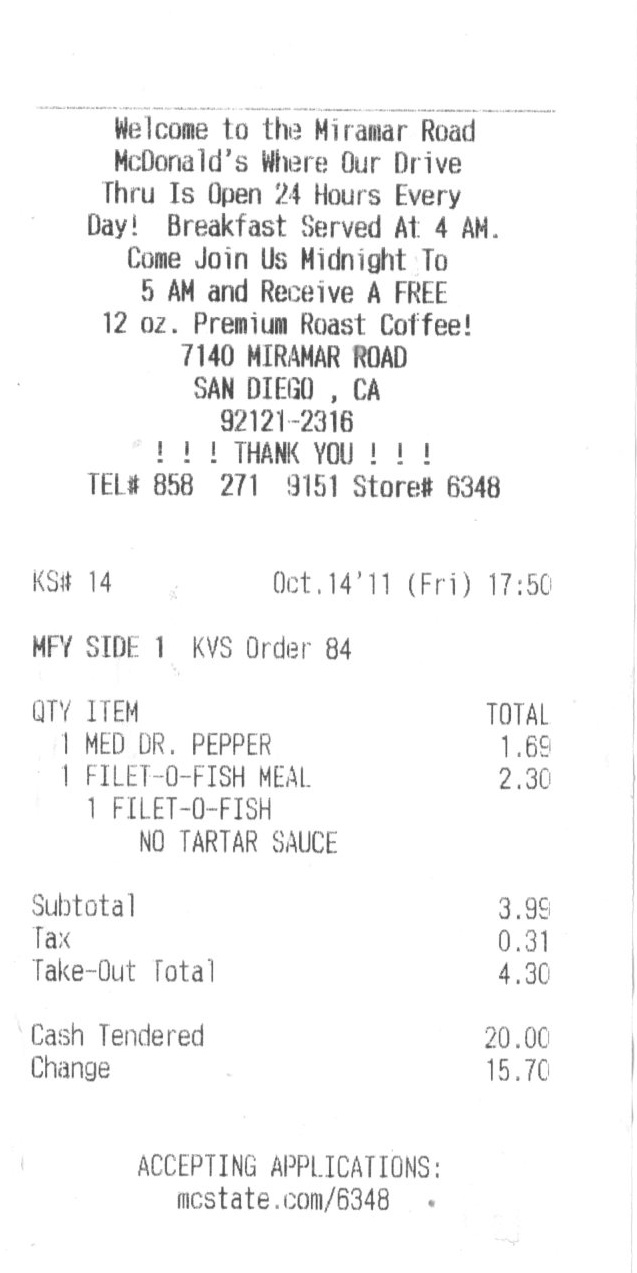The black and white image appears to be a scanned photocopy of a McDonald's receipt from the Miramar Road location in San Diego, California. The receipt's header welcomes customers to the McDonald's at 7140 Miramar Road, highlighting that their drive-thru operates 24 hours every day, with breakfast service starting at 4 a.m. Additionally, it invites patrons to visit between midnight and 5 a.m. for a free 12-ounce premium roast coffee. 

The receipt lists the store number (6348) and contact information (telephone number 858-271-9151) followed by the details of the order. The transaction includes one medium Dr. Pepper priced at $1.69 and a Filet-O-Fish meal costing $2.30, specifically noted to be without tartar sauce. The subtotal amounts to $3.99, with an additional tax of $0.31, bringing the takeout total to $4.30. The payment was made with a $20 bill, resulting in $15.70 as change.

At the bottom, the receipt indicates that the McDonald's store is accepting job applications, directing potential applicants to the website McState.com/6348. The message of gratitude is emphasized with three exclamation points.